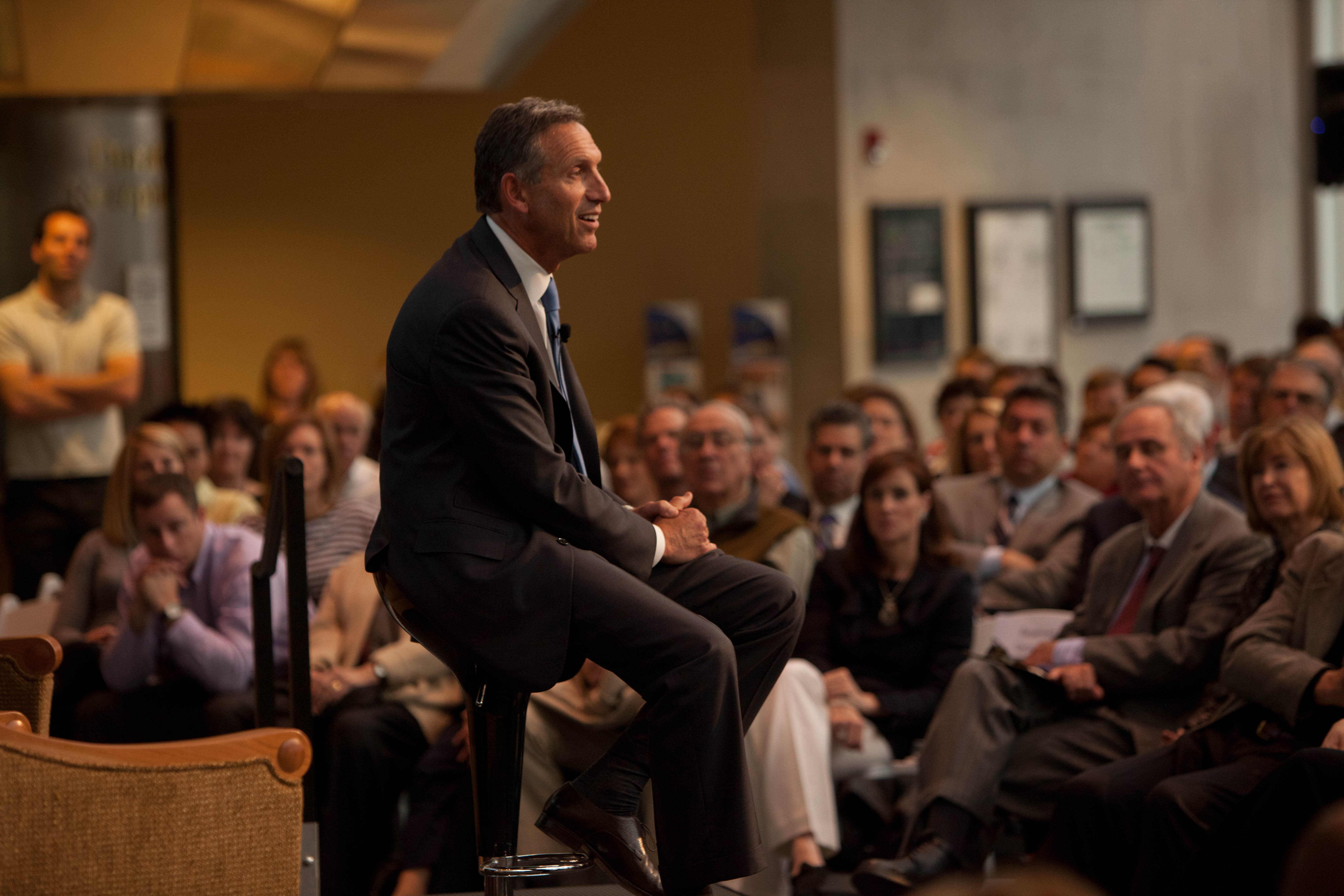In a well-composed, professional photograph, an older white man in his 60s, dressed in a gray suit with a white shirt and light blue tie, is seated on a small black stool at the center of a large room. A discreet microphone is clipped to his tie. He is the focal point of the image, captured mid-speech, addressing an attentive audience comprising men and women of various ages. The attendees are engrossed in his presentation, sitting quietly in rows, except for one man standing towards the far left with his arms crossed. The background reveals a large room with light brown and white walls adorned with three plaques. The color palette of the scene includes various shades of brown, yellow, beige, black, white, gray, blue, some silver, and pink. Additional details include another chair, likely wooden with brown upholstery, positioned behind the speaker. The photograph's clarity and angle suggest it was taken by a professional, capturing the seriousness and focus of the event.